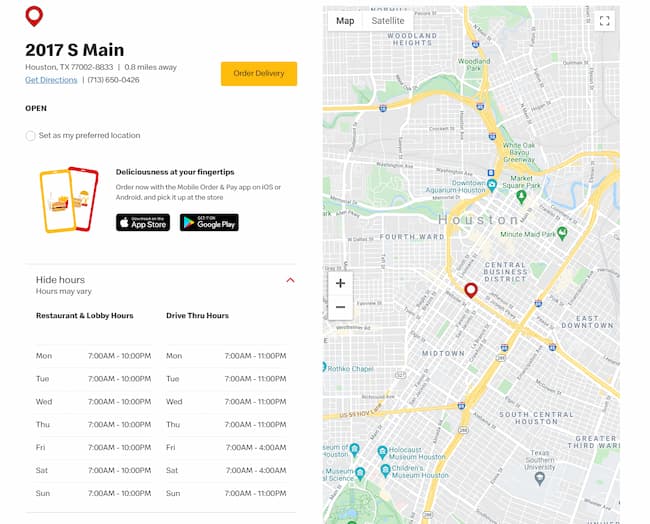This cropped image from a restaurant’s order delivery section on their website prominently features a dual-section display. The image is neatly divided into two halves, with the left side showcasing essential restaurant information on a clean white panel and the right side depicting a detailed map with a pin indicating the restaurant's precise location.

On the left panel, a pin drop icon is positioned at the top, followed by the restaurant’s address, "2017 South Main," in bold black font for emphasis. Below the street address, the city, zip code, and distance are provided in regular text. A hyperlink reading "Get directions" is situated to the left, while the restaurant's phone number is conveniently displayed to the right. Further down, the word "Open" is highlighted in small, bold black letters, and beneath it, there is an option to set this location as your preferred one, marked by a clickable dot.

An inviting advertisement follows, proclaiming "Deliciousness at your fingertips. Order with the mobile order and pay app on iOS or Android and pick it up at the store." This call-to-action is accompanied by two icons for the Apple App Store (left) and Google Play Store (right), facilitating easy app downloads.

The lower section of the panel features operational hours. A "Hide hours" option is located on the left, with a dropdown menu on the far right to collapse this section if desired. Below, the operation hours are split into two categories: "Restaurant and Lobby Hours" on the left and "Drive-thru Hours" on the right, each followed by a vertical list of their respective times, clearly outlining the hours of service.

The entire right side of the image is dedicated to a visually appealing map, complete with a pin drop marking the restaurant's location, providing users with a clear geographic reference point.